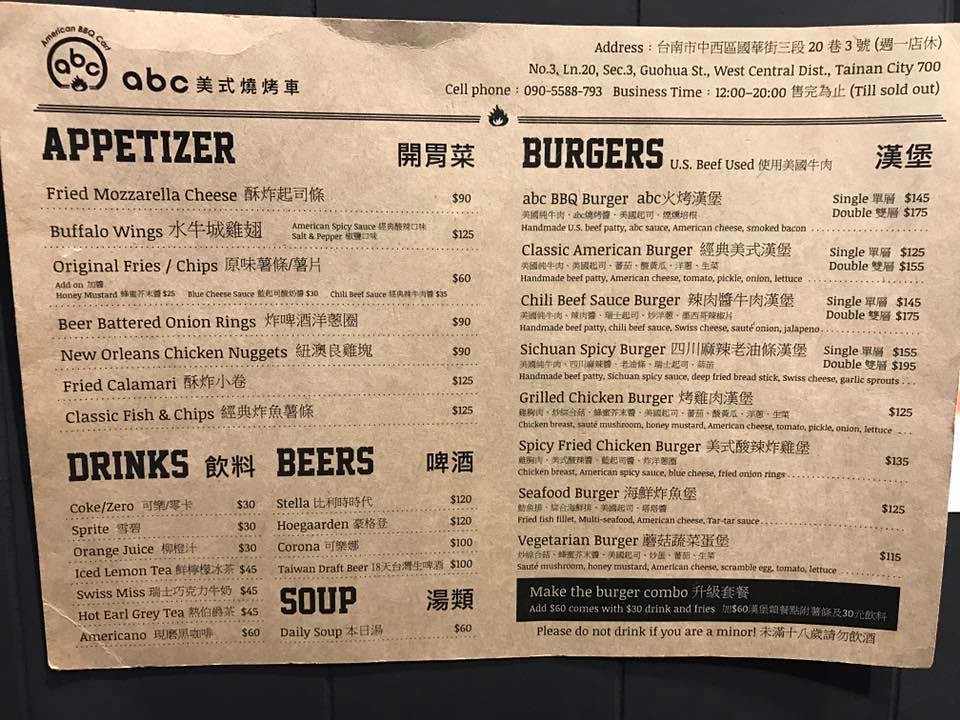A well-worn and slightly dingy restaurant menu, featuring both English and an East Asian language—possibly Japanese or Chinese. The menu offers a variety of American-style dishes, including fried mozzarella cheese sticks, buffalo wings, and various soups. Beverage options include soft drinks and a selection of beers. The menu is divided into sections: Appetizers, Drinks, Beers, Soups, Burgers, and a special American Barbecue section. It also highlights a "Build Your Own Burger" option, with choices such as beef, chicken, seafood, and vegetarian burgers. A note at the bottom advises patrons against underage drinking. The menu lists the restaurant’s address and phone number at the top.